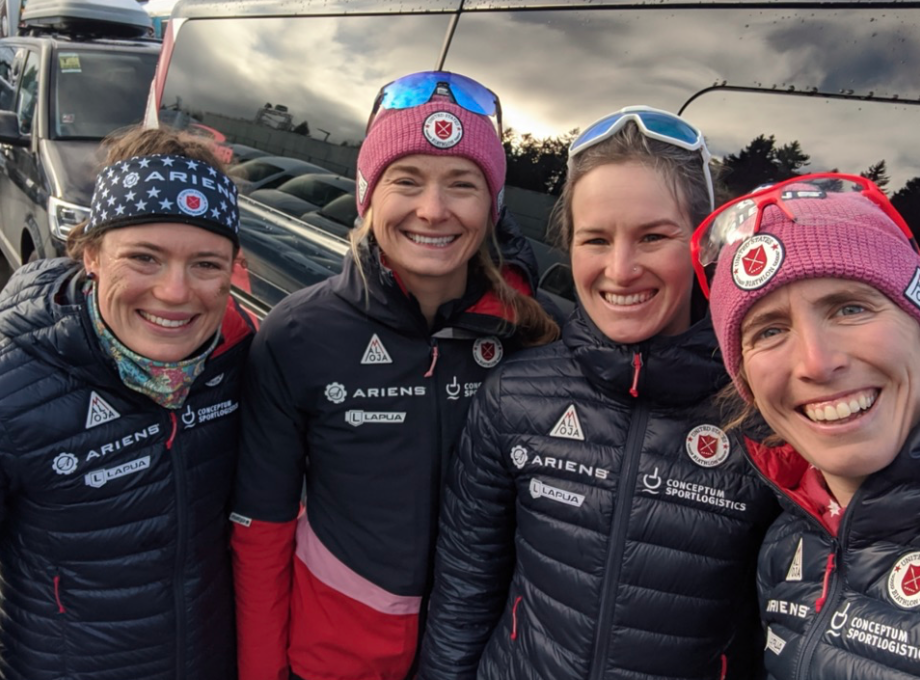This photograph captures an enthusiastic group of four women, all donning stylish winter gear, standing in front of a sleek and shiny black van. Each woman is wearing a matching black winter jacket emblazoned with a triangular "Ariens" logo at the bottom and a circular logo with a red crest and small text on the right side. Their headgear varies, with the woman on the far left sporting a navy blue bandana featuring the "Ariens" logo and the others wearing pink beanies. The second woman from the left has perched sunglasses on her head, while the third woman wears blue sunglasses with a white frame. The woman on the right, wearing a similar pink beanie, has red-framed glasses on her head. All four women exude joy, their smiles wide and bright, suggesting they are likely enjoying a ski vacation or outdoor winter adventure. The background shows daylight reflecting off the vehicle, with another van visible in the distance, enhancing the scene's overall vibrant and lively atmosphere.